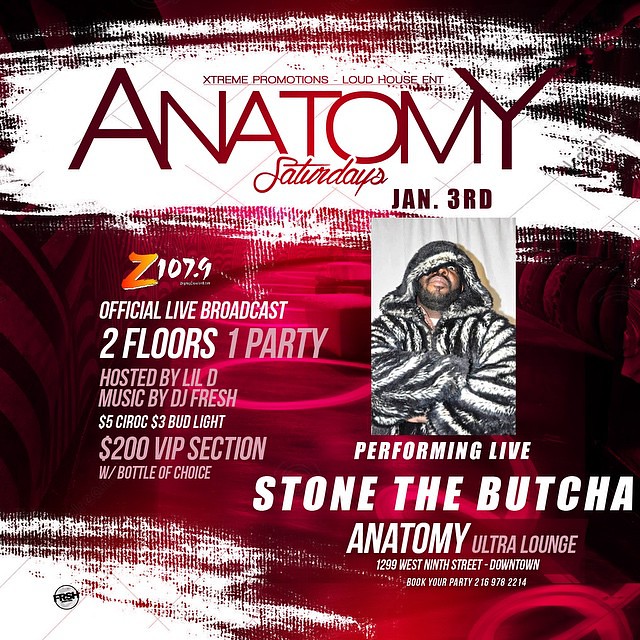The poster is an eye-catching advertisement for a live performance event titled "Anatomy Saturdays," set to take place on January 3rd. Promoted by Extreme Promotions, Loud House Entertainment, and ENT, the event promises an exciting night hosted by Lil D. The title "Anatomy Saturdays" is prominently displayed at the top in bold red text, flanked above by "Extreme Promotions, Loud House," and below by the date, January 3rd.

On the left side of the poster, detailed information about the event is provided. It mentions an official live broadcast by Z100, featuring two floors of music with DJ Fresh. Partygoers can enjoy drink specials such as $5 Seek Road and $3 Bud Light, with a $200 VIP section that includes a bottle of choice.

On the right side of the poster, there is a striking image of a man wearing a luxurious grey and white fur coat and hat, sporting a black mustache and beard along his jawline. Below this image, the text announces the live performance by "Stone the Butcher," along with "Anthony" and "Ultra Lounge."

Additional details are included at the bottom of the poster, such as contact information, addressing 1299 West 9th Street, downtown, and a phone number for booking: 216-978-2214. The background of the flyer features abstract red and pink patterns, enhancing its vibrant and dynamic visual appeal.